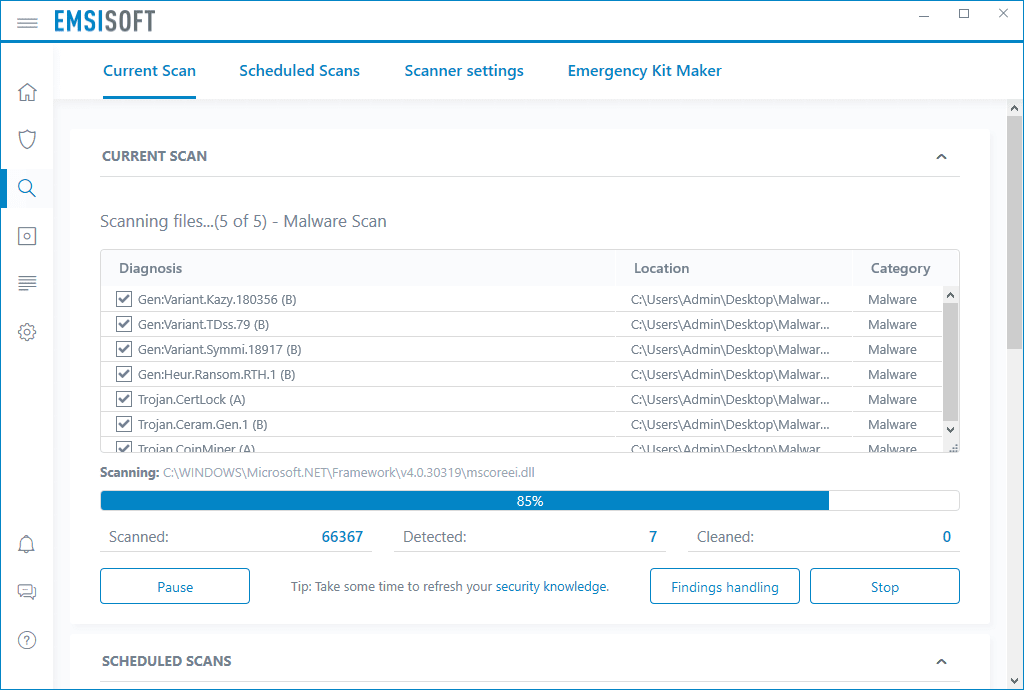Screenshot of Emsisoft Anti-Malware Scan Interface

The screenshot displays the interface of the Emsisoft anti-malware software. At the top left corner, three horizontal lines representing the menu icon are present. Directly to the right, the brand name is clearly visible, with "EMSI" in bold blue letters and "SOFT" in gray letters. On the top right corner, the standard window control buttons – minimize, reduce, and close (X) – are visible.

Below the top section, the interface prominently indicates the status of the current scan. The "Current Scan" label is in dark gray, followed by "Scanning files... 5 of 5 - Malware Scan" in lighter gray. This section appears to be the scanning progress overview.

Further down, there is a section labeled "Diagnosis" in dark gray. Adjacent to this, columns are labeled "Location" and "Category." The list below includes various detected threats, each with a gray check mark inside a white box, indicating identified malware. The details for each entry are as follows:

1. **Gen Variant KZ.18356B**
   - **Location:** C:\Users\Admin\Desktop\Malware (truncated)
   - **Category:** Malware

2. **Gen Variant TDSS.79B**
   - **Location:** C:\Users\Admin\Desktop\Malware
   - **Category:** Malware

3. **Gen Variant.SYMMI.18917B**
   - **Location:** C:\Users\Admin\Desktop\Malware
   - **Category:** Malware

4. **Gen:HEUR.ransom.RTH.1B**
   - **Location:** C:\Users\Admin\Desktop\Malware
   - **Category:** Malware

5. **Trojan.certlockA**
   - **Location:** C:\Users\Admin\Desktop\Malware
   - **Category:** Malware

6. **Trojan.CERAM.GEN.1B**
   - **Location:** C:\Users\Admin\Desktop\Malware
   - **Category:** Malware

At the bottom part of the interface, a blue button displays "85%" in white text, indicating the progress of the scan. Just above this button, the word "Scanning" is noted, reflecting the ongoing action.

Overall, the screenshot provides a detailed view of the Emsisoft anti-malware scan results, showcasing various detected threats alongside their file locations and classifications.